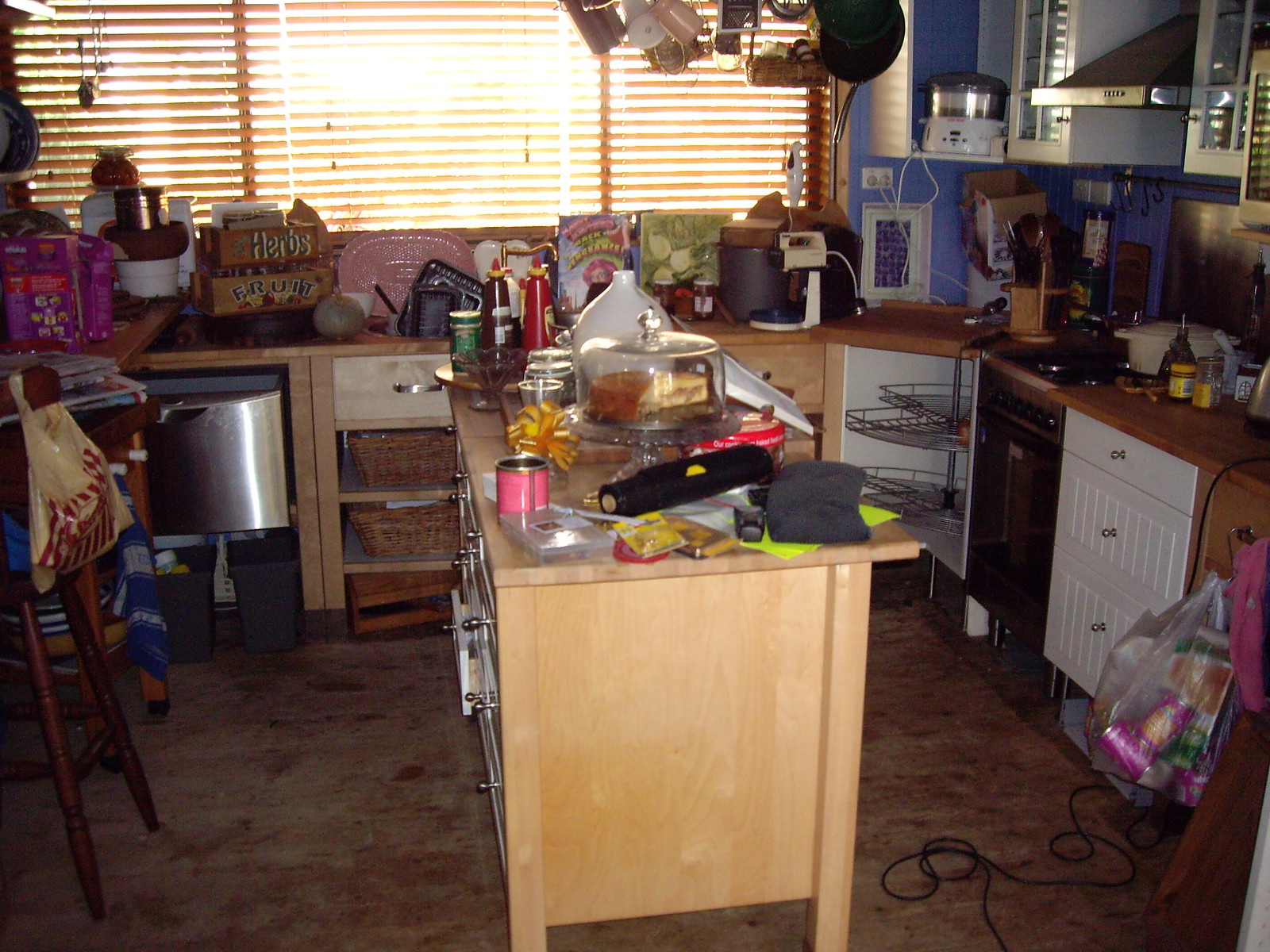A dimly lit kitchen, primarily illuminated by sunlight streaming through a large window adorned with brown blinds, is bustling with various items and details. At the heart of the room stands a light wooden island, cluttered with a half-eaten cake encased in a glass dome, a single glove, miscellaneous papers, and a large bottle—perhaps vinegar. Further down is a rack filled with additional items. The island features drawers with silver handles.

Surrounding the island, expansive counter space stretches around the kitchen. To the far left, one can spot a trash can with a silver metallic drawer, a small appliance on the counter, and a hint of a stool with a grocery bag hanging from it. Nearby, the sink area is somewhat chaotic with a pan and various other items, accentuated by a glimpse of a gold faucet.

Continuing right along the counter, more assorted items are visible. The stove area, highlighted by a black overhead and a blue-painted wall, stands out. An overhead cabinet, partially open, reveals a cooker, while pots and pans dangle from the ceiling. On the stove, a Dutch oven takes center stage, below which a Lazy Susan in the base cabinet appears empty.

Adjacent to the stove, three drawers and another countertop hold several items, including a clear plastic grocery bag filled with cans, hinting at potential recycling, alongside a small pink towel. An errant black cord snakes across the floor, perhaps connected to an unseen appliance. This vivid tableau offers a snapshot of a busy, well-used kitchen brimming with life and activity.